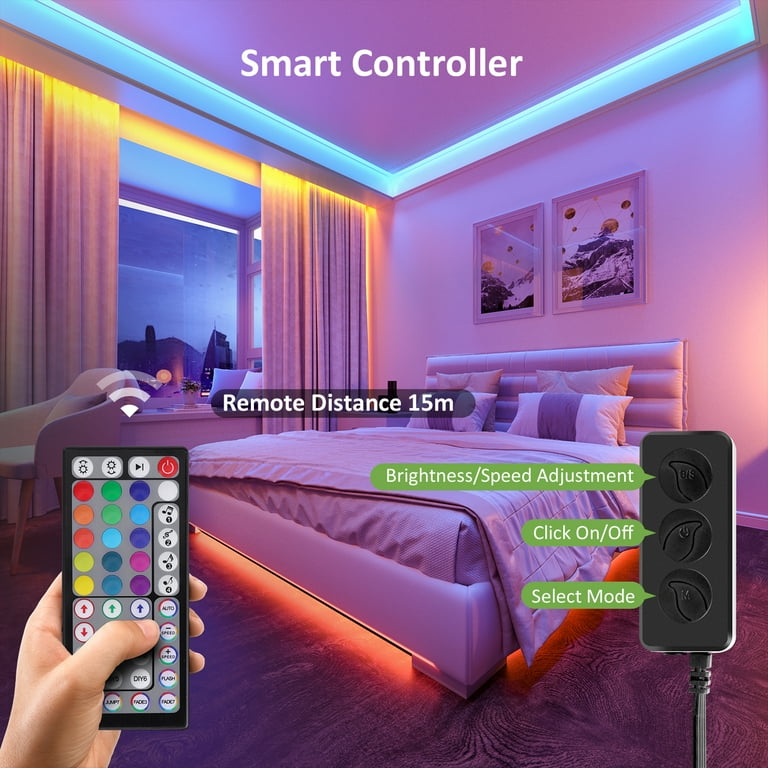The photograph is a highly detailed advertisement showcasing the operation of a smart controller for a lighting fixture in a modern bedroom. The room features a large bed with a white bedspread and two picture frames hanging above the headboard. There's a large window with curtains, adding to the sleek, contemporary design.

The image is bathed in vibrant, colorful lighting, ranging from purple to blue to yellow, with an orange glow emanating from under the bed and a soft baby blue light outlining the top of the ceiling. "Smart Controller" is prominently displayed in large white text across the top of the image, emphasizing the focus of the advertisement.

In the bottom left corner, a hand holds a smart controller device equipped with numerous buttons, including colorful ones that control the light's colors, brightness, and speed. An additional controller is visible on the right side, featuring buttons for on-off functions, brightness, speed adjustment, and mode selection. Notably, this device also includes various icons, such as arrows and musical notes, indicating multifunctional capabilities. In the center of the image, small white text states, "Remote distance 15 meters," suggesting the effective operational range of the smart controller.